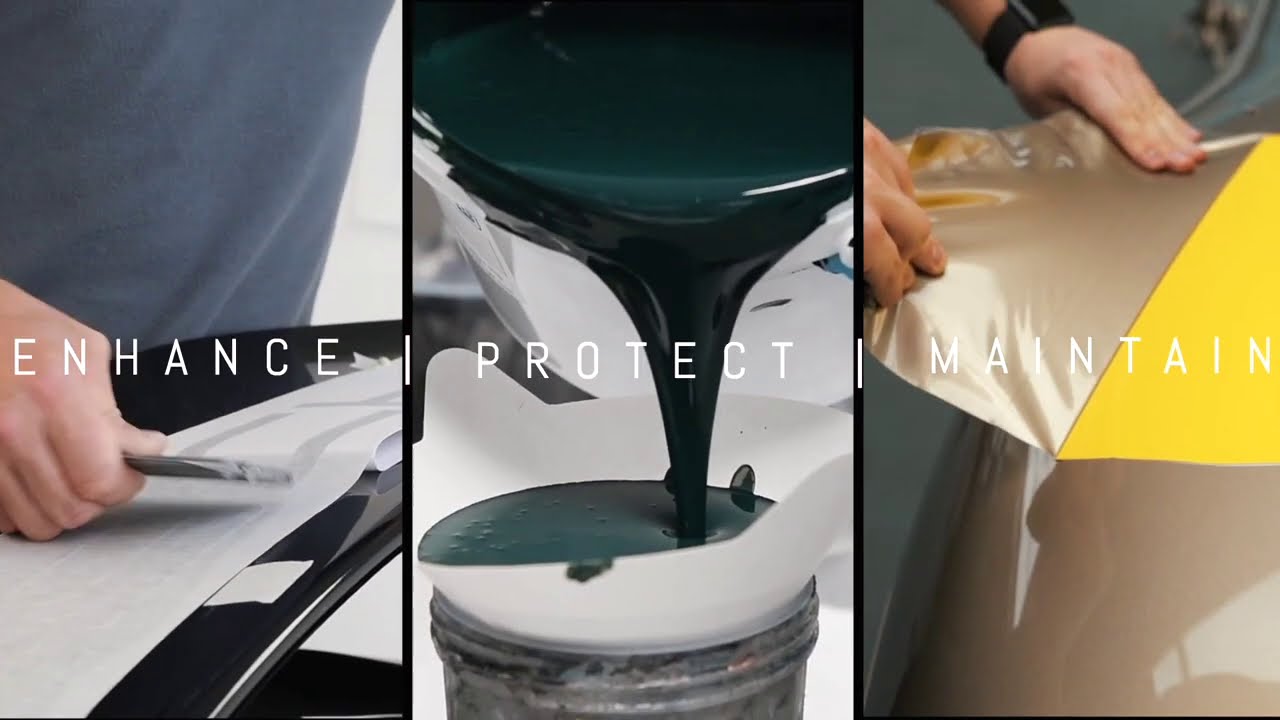The image is a horizontal rectangular graphic art divided into three vertical segments, each showcasing close-up photographs with the words "Enhance," "Protect," and "Maintain" in bold white capital letters. 

In the left panel, labeled "Enhance," there is a close-up of a person in a blue shirt using a tool to map out something on a piece of white material over a black surface, possibly working on a glossy curved object.

The middle panel, labeled "Protect," features dark green paint being poured from a bucket into another container, suggesting the careful preparation or application of materials, possibly in a protective coating process.

The right panel, labeled "Maintain," shows hands, one wearing a watch, meticulously sewing or assembling a golden-beige fabric or material over a grayish-brown object.

This image appears to be a promotional graphic for a craft or manufacturing company, illustrating the processes involved in enhancing, protecting, and maintaining products.